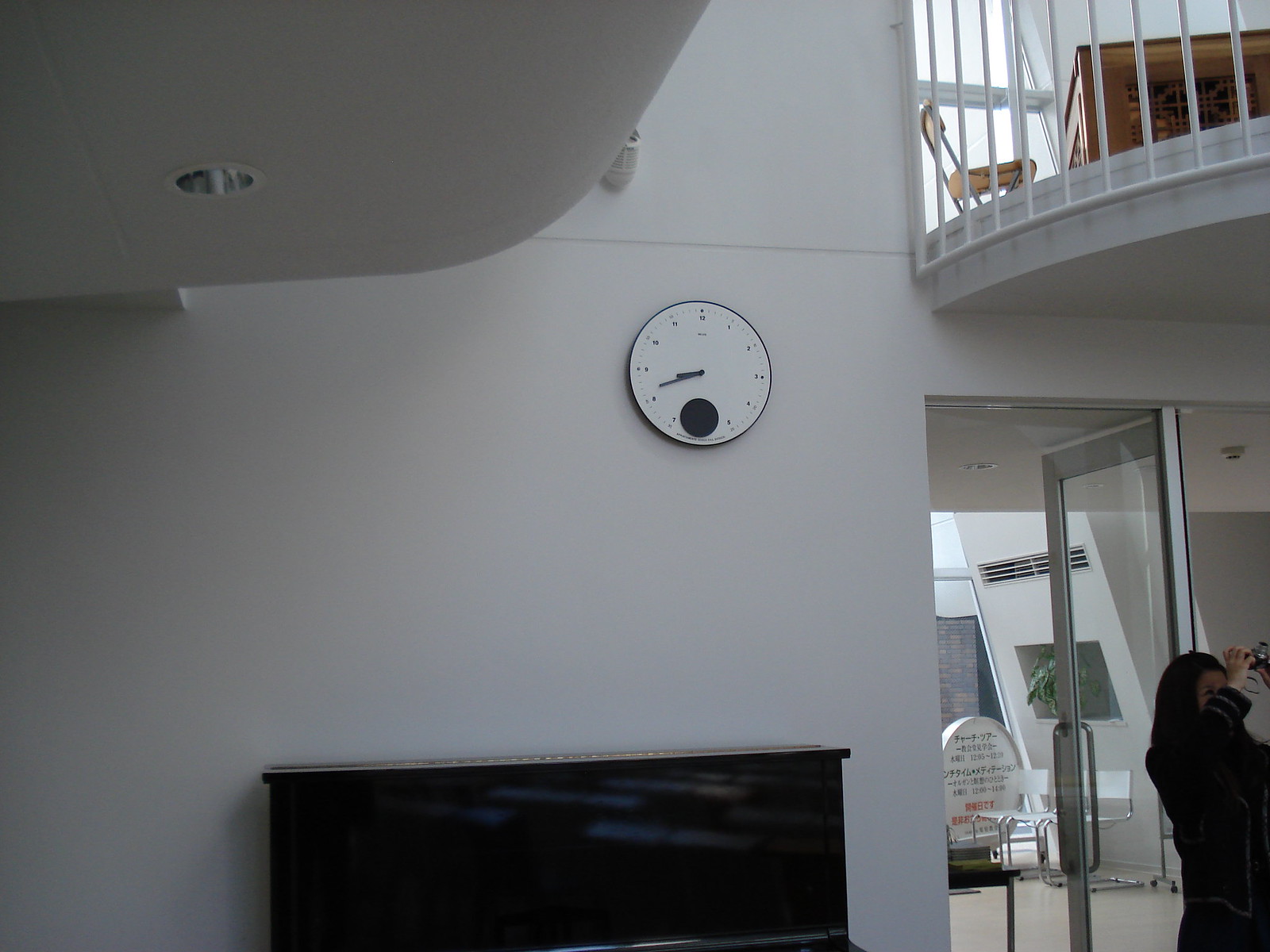The photograph depicts an art museum or gallery, characterized by its modern architectural design and open event space. The pristine white walls provide a clean backdrop, enhancing the minimalist aesthetic. A sleek clock adorns one of the walls, featuring a white face, round shape, small black numbers, and a very thin black rim with black hands. A glass entrance door, framed in metal with a typical handle, can be seen towards the right in the background. This leads to a reflective black piano, which adds a touch of elegance to the scene. On the left, an upstairs balustrade is visible, along with a desk and chair, suggesting office or administrative use. Abundant natural light floods the space through numerous windows, creating a bright and inviting atmosphere. In the foreground, a woman dressed in black stands by the entrance, capturing a photograph of something above her with a handheld camera, adding a dynamic element to the serene setting.